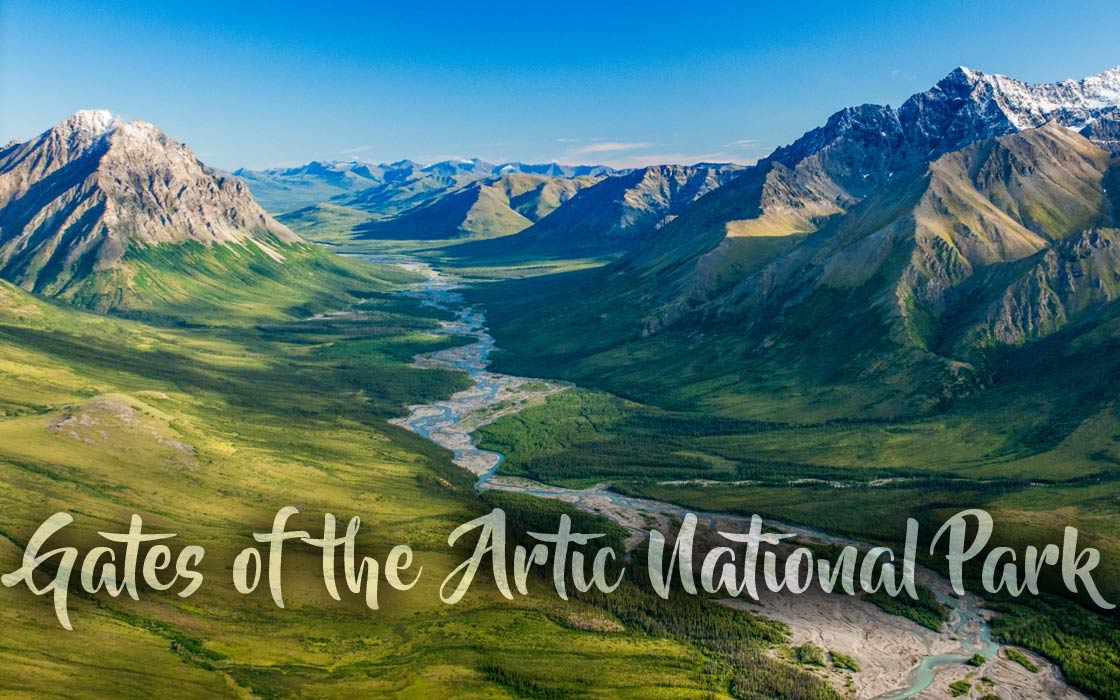The picture, resembling a postcard or poster, showcases a breathtaking, wide-shot view of the Gates of the Arctic National Park, a serene and untouched natural landscape. The expansive image, bathed in daytime light, is dominated by a sprawling, verdant valley nestled between towering mountain peaks. In the central focus, a winding river courses through the valley, bordered by sandy banks that contrast with the lush greenery. The river's water appears tinged with sediment, maintaining a natural, rugged appearance. Framing the scene, the mountains rise majestically on either side, their gray peaks dusted with patches of snow, hinting at the Arctic chill. Overhead, the sky stretches wide and clear, with no clouds disrupting the vivid blue expanse. The title, "Gates of the Arctic National Park," is elegantly scripted across the bottom in a relaxed white cursive font, perfectly complementing the tranquil yet awe-inspiring beauty of the landscape.